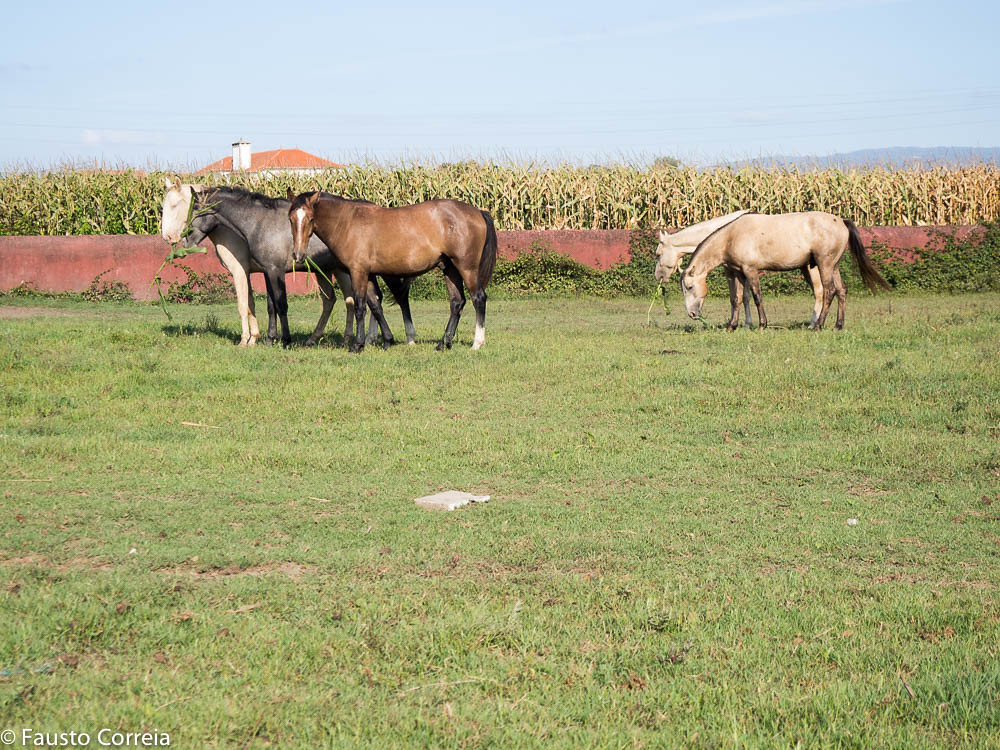In the image, five horses are seen grazing peacefully in an open, well-manicured grassy field on a ranch. Among the horses, three are whitish, one is black, and one is brown with a distinctive white stripe on its head and white markings on its rear legs. One of the horses appears to be glancing towards the camera, while the rest are looking off to the side. In the background, a tall crop field, possibly corn, stands behind a short brick wall that separates it from the grassy area. Beyond the cornfield, a house with a red roof and a white chimney is just visible, set against what looks like a large hill or mountain under a partly cloudy blue sky. The bottom left corner of the image features a copyright notice: "© Fausto Correa."